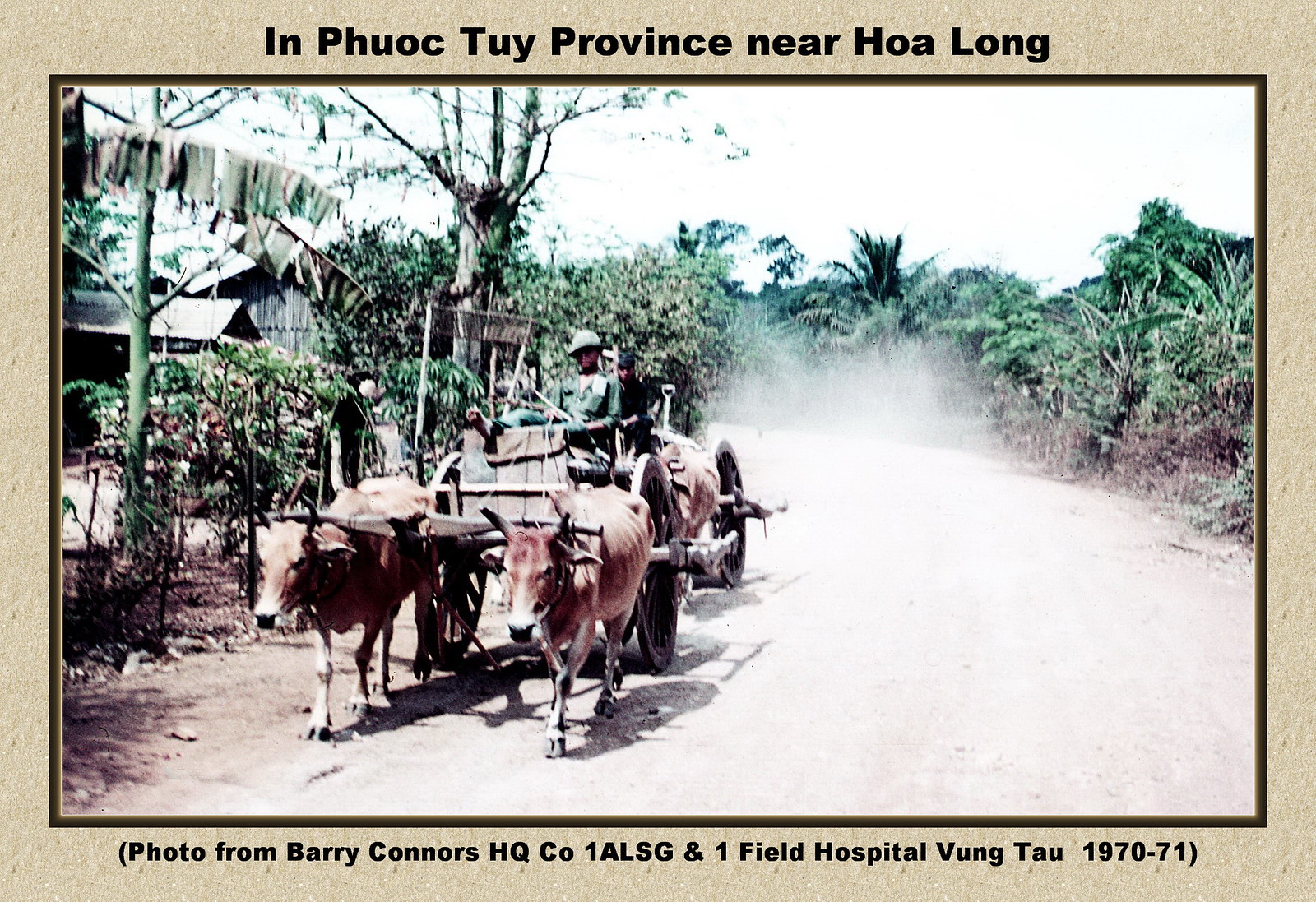This color photo from 1970-1971 captures a scene in Phước Tuy province near Hòa Long, Vietnam, as noted in the caption and the border itself on the image. The caption at the bottom credits Barry Connors, HQ CO1 ALSG, and One Field Hospital Vũng Tàu. The image depicts an ox-drawn cart made out of wood, with large wheels on both sides, navigating a dusty dirt road. The cart is being pulled by two brown oxen, not donkeys or horses as initially speculated. Seated on the cart is a man wearing a hat, likely a military personnel given the context. To the right, there are tropical trees and maybe tents, while to the left appears to be a farm-like wooden structure. The background is filled with tropical foliage, creating a lush green contrast against the dusty road, which kicks up a cloud of dust as the cart moves. The sky above is mostly white and saturated. The image itself is bordered by an earth-toned, brownish frame that adds to the vintage feel.